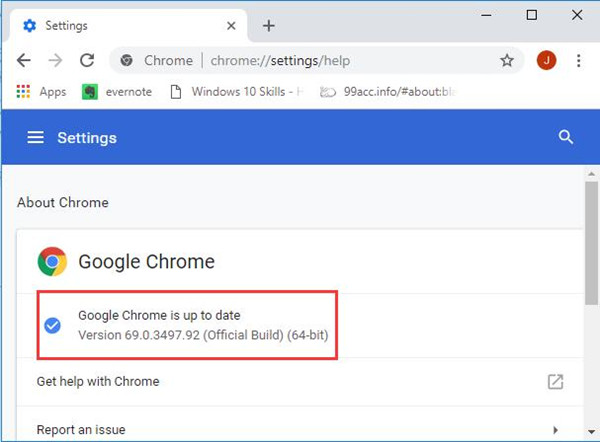This is a detailed screenshot of a Google Chrome settings page on a computer. In the upper-left corner, the word "Settings" is prominently displayed. Below it, there is a small blue bolt symbol. Moving downward, there are navigation icons including a left arrow, a right arrow, and a refresh arrow.

The interface features the words "Chrome," "Chrome settings," and "Help." A large blue bar spans the screen with the word "Settings" prominently in the middle. To the right of this bar, there's a magnifying glass icon indicating a search functionality. 

Beneath the blue bar, the heading "About Chrome" appears. Under this heading is the recognizable Google Chrome logo, a circle segmented into four colors: red, green, yellow, and blue, featuring the phrase "Google Chrome." Below the logo, there is a red box containing a blue circle with a checkmark, accompanied by the text "Google Chrome is up-to-date." It specifies the version as "Version 69.0.3497.92 (Official Build) (64-bit)."

Further down, options to "Get help with Chrome" and "Report an issue" are available. To the right side of the screen, the vertical scrollbar is visible, indicating that the page content can be navigated up and down. This screenshot captures a user viewing their Google Chrome settings, specifically checking for updates and confirming their browser is up to date.